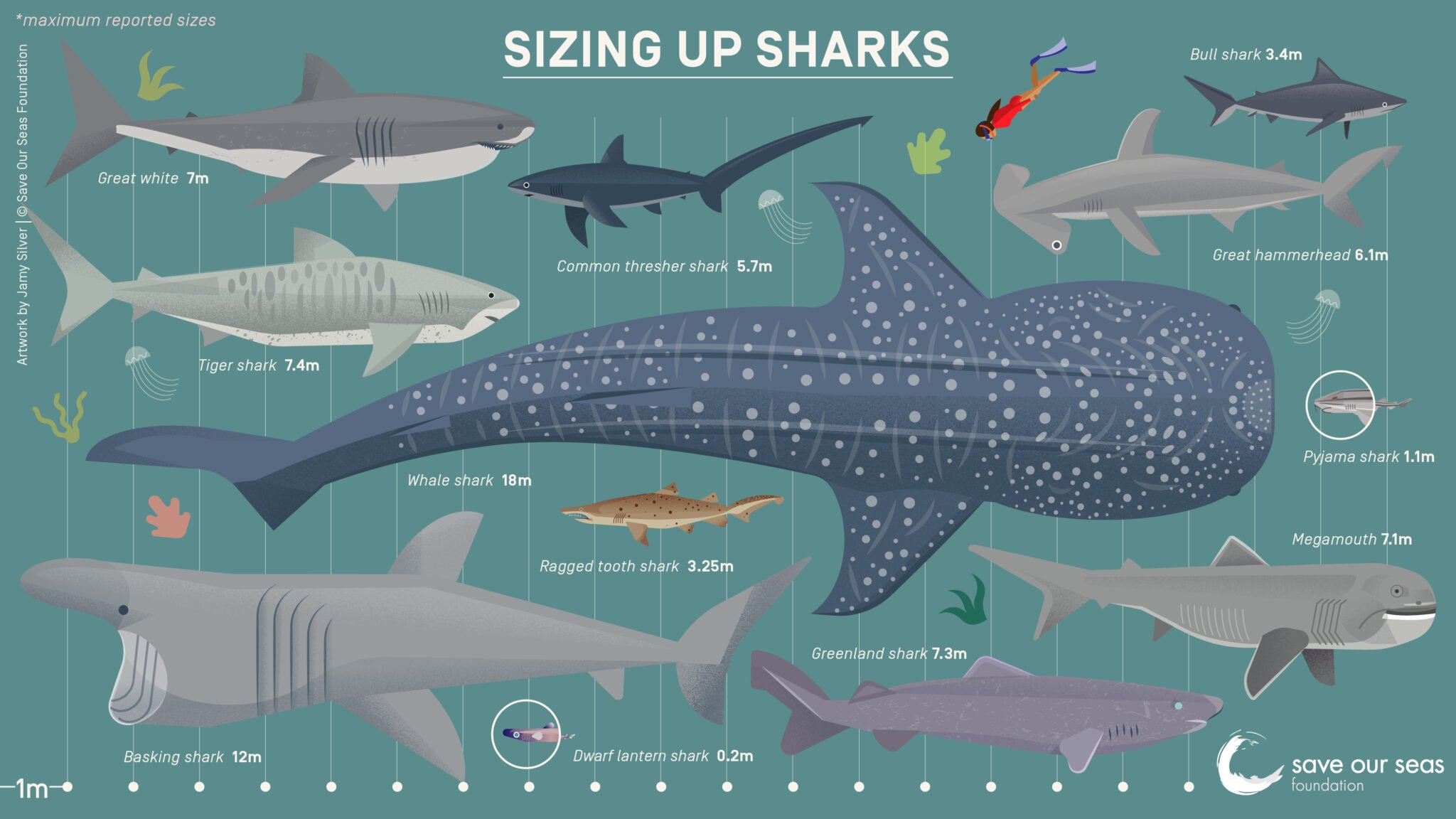This detailed illustration compares the sizes of various shark species against a human diver for scale. At the upper center right, a female diver with dark hair is depicted wearing a red short wetsuit and blue fins, providing a clear reference for the relative sizes of the sharks. 

Dominating the chart is a whale shark, illustrated at an impressive length of 18 meters, facing right. The whale shark is characterized by its gray body adorned with white spots, excluding its tail.

In the upper left corner, a great white shark is shown, labeled "7M." Below it is a tiger shark marked at 7.4 meters, and further down, a basking shark is depicted, stretching out to 12 meters.

On the right side of the image, several other shark species are illustrated:
- A great hammerhead measuring 6.1 meters.
- A bull shark at 3.4 meters.
- A megamouth shark at 7.1 meters.
- A Greenland shark at 7.3 meters.

The center of the image prominently features the title "Sizing Up Sharks" in white lettering. The entire illustration is set against an aqua green background, with all textual elements standing out in white.